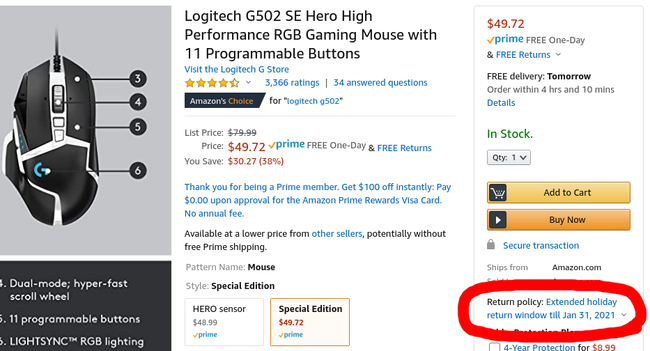This detailed caption describes the image clearly:

The image is a partial screenshot from an Amazon.com product page for a Logitech mouse. The image is cropped, cutting off portions of the top, left-hand side, and bottom. On the visible left side of the image, there is a picture of the product: a black Logitech mouse with silver sections. Adjacent to the picture is the product name in large, bold black text: "Logitech G502SE Hero High Performance RGB Gaming Mouse with 11 Programmable Buttons." Beneath this text, there is a blue hyperlink that says "Visit the Logitech Store." Further down, the list price of $79.99 is struck through, and the actual price is shown as $49.72 with Amazon Prime benefits. Customers can choose between two options: the Hero Sensor Version or the Special Edition, with the Special Edition highlighted.

On the right-hand side of the screenshot, there is another column containing additional purchase-related information. A section is emphasized with a red circle, added later to draw attention to specific text. The highlighted text states the return policy: "Extend the holiday return window till January 31st, 2021."